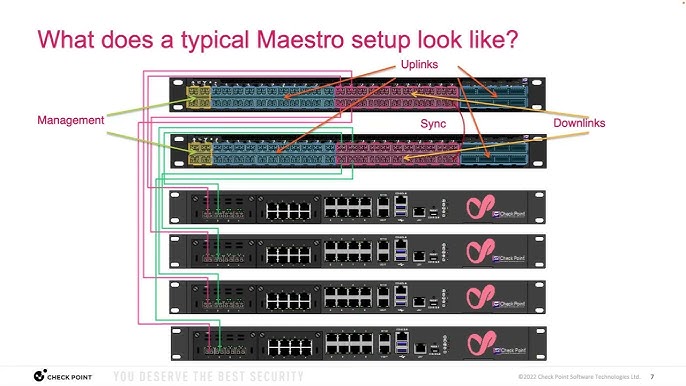The image depicts a detailed diagram of a typical Maestro setup against a white background. At the top, bold magenta text asks, "What does a typical Maestro setup look like?" Below this, the diagram is divided into several sections. The first two sections are nearly identical, featuring black bars labeled with various components essential for the setup: "uplinks," "management," "sync," and "downlinks." Each of these labels is accompanied by colored arrows pointing to specific ports, indicating their respective functions. The third section displays four identical electronic devices viewed from the back, showing where various connections such as USB and Ethernet ports are located. Green and purple lines further highlight these points of connection. At the bottom left of the image, there is a logo reading "Checkpoint," followed by the slogan, "You deserve the best security." In addition, black bars with multicolored sections illustrate different levels of menus or configurations, providing a comprehensive visual guide.